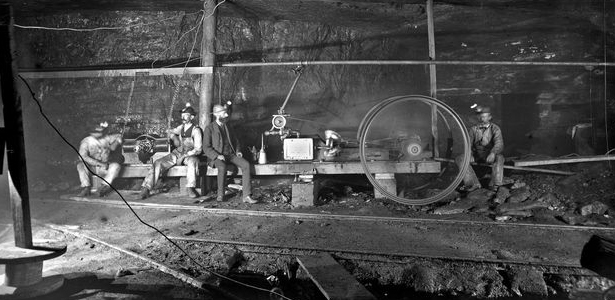This detailed black and white photograph, likely taken around a hundred years ago, depicts four men resting in what appears to be a mine shaft. The horizontally oriented image captures the men sitting on a wooden bench surrounded by various materials and equipment. They are dressed in work outfits, with some wearing miner's helmets that have lights turned on, illuminating their faces against the darker right side of the image. 

In the background, there is a large, imposing black wall supported by wooden beams, reinforcing the underground setting. The foreground is littered with dirt and wooden planks. Toward the right side of the bench, a large, indistinct spinning wheel—possibly a piece of machinery—adds to the industrial atmosphere. Light streams in from the left, casting shadows and highlighting the weathered, resigned expressions of the men, who appear to have paused their labor. Their diverse clothing, ranging from dirty work clothes to one darker suit, underscores their varying roles in this rugged environment.

Overall, the photograph's historical vibe is enhanced by the visible wear on the men's clothing and the antiquated equipment, transporting the viewer to an early 20th-century mining operation.